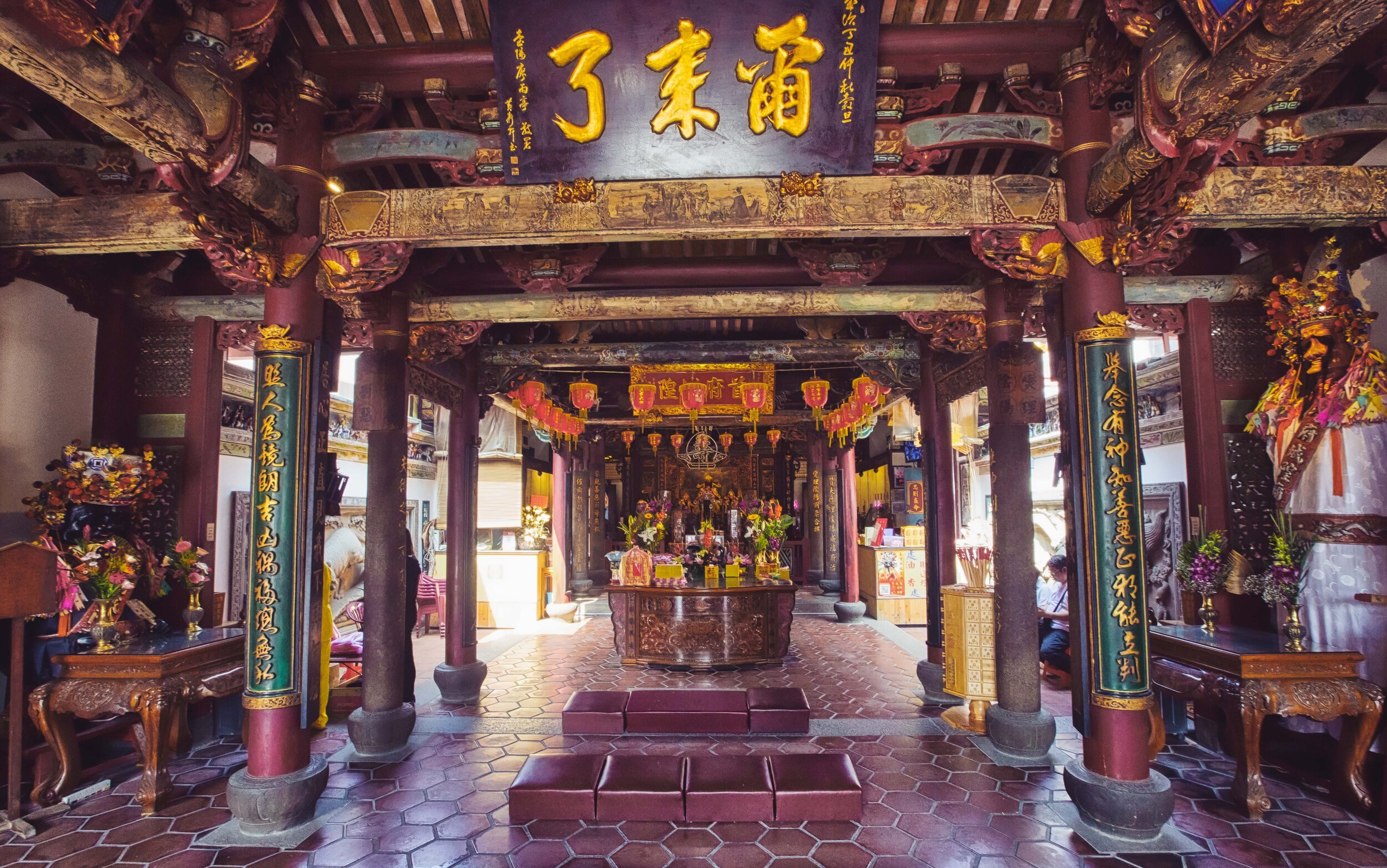The photograph depicts a traditional Asian, likely Chinese, establishment that could be a temple or a market. The scene is richly detailed and ornate, featuring a series of wooden archways adorned with green signs with vertical foreign lettering likely in Chinese characters. Red paper lanterns hang from the ceiling, adding a vibrant touch. The archways, supported by large red pillars, lead the viewer's eye down a central path. The maroon hexagonal-tiled floor contrasts with the wooden structures. At the end of the archway, a table decorated with various plants and flowers can be seen, hinting at an altar or display area. Both sides of the path are lined with tables showcasing dried flowers and vases, which introduce a serene, decorative element. The establishment appears to be semi-outdoor, with sunlight filtering through openings that seem to lead to other rooms or sections. The overall color palette includes deep maroons and purples, complemented by green and gold lettering, creating a traditional, visually captivating ambiance.